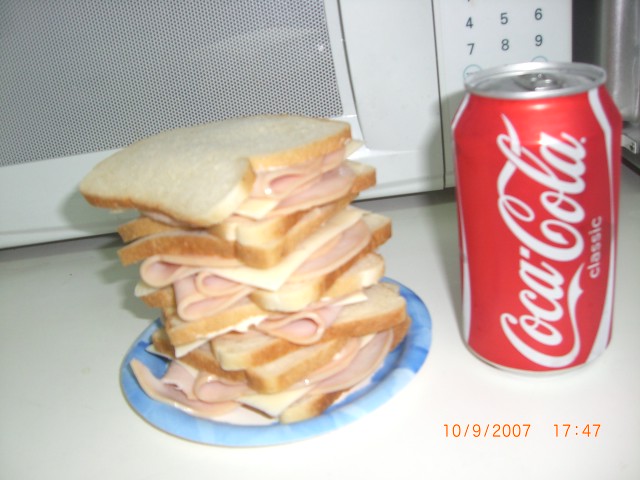The image depicts a white countertop with a white microwave featuring a white keypad with black numbers. In the foreground, there's a blue paper plate, which has a mix of dark and light blue hues with white accents. On the plate are four sandwiches made with white bread, showing a light brown crust edge. The sandwiches are haphazardly stacked, with filling comprising lunch meat that has a pinkish hue, resembling either turkey or bologna, paired with a light yellow cheese, possibly Swiss. Alongside the plate, there is an unopened red and white Coca-Cola can with a silver top, displaying the classic "Coca-Cola" logo in white. The image also includes a timestamp located in the bottom right corner, showing the date as 10-9-2007 and the time as 17:47. A shadow is noticeable beneath the microwave and to its left, adding depth to the setting.